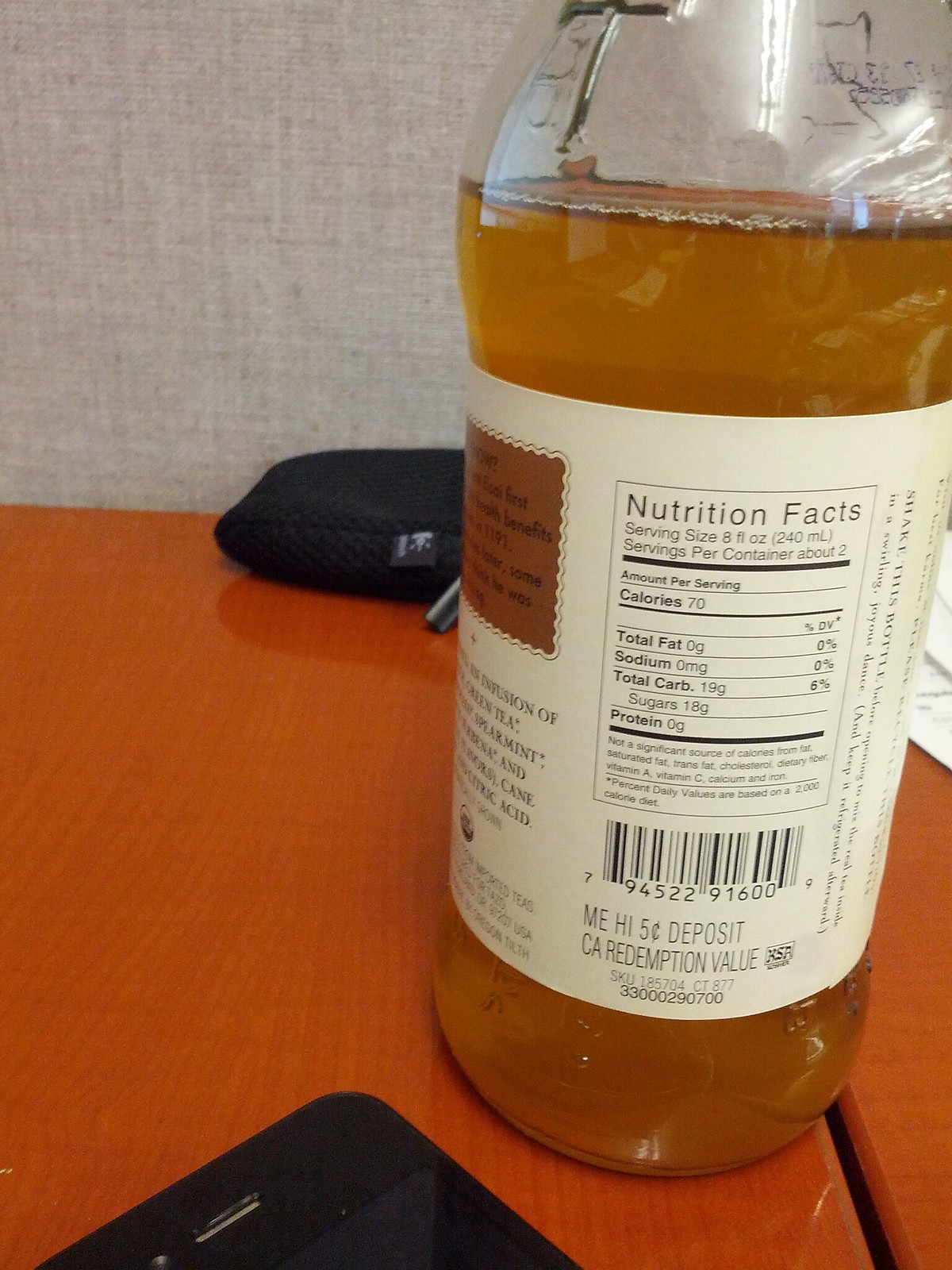The photograph captures a moment during a school break, focusing on a juice container with detailed nutritional facts. The container highlights that an 8-fluid ounce serving has approximately 70 calories, 0 total fat, 0 sodium, 19 grams of total carbohydrates, and 18 grams of sugar. Below the juice container, there is also a phone placed, adding a modern, everyday touch to the scene. The overall atmosphere suggests an ordinary school day with an emphasis on the nutritional information of the beverages consumed by the students.